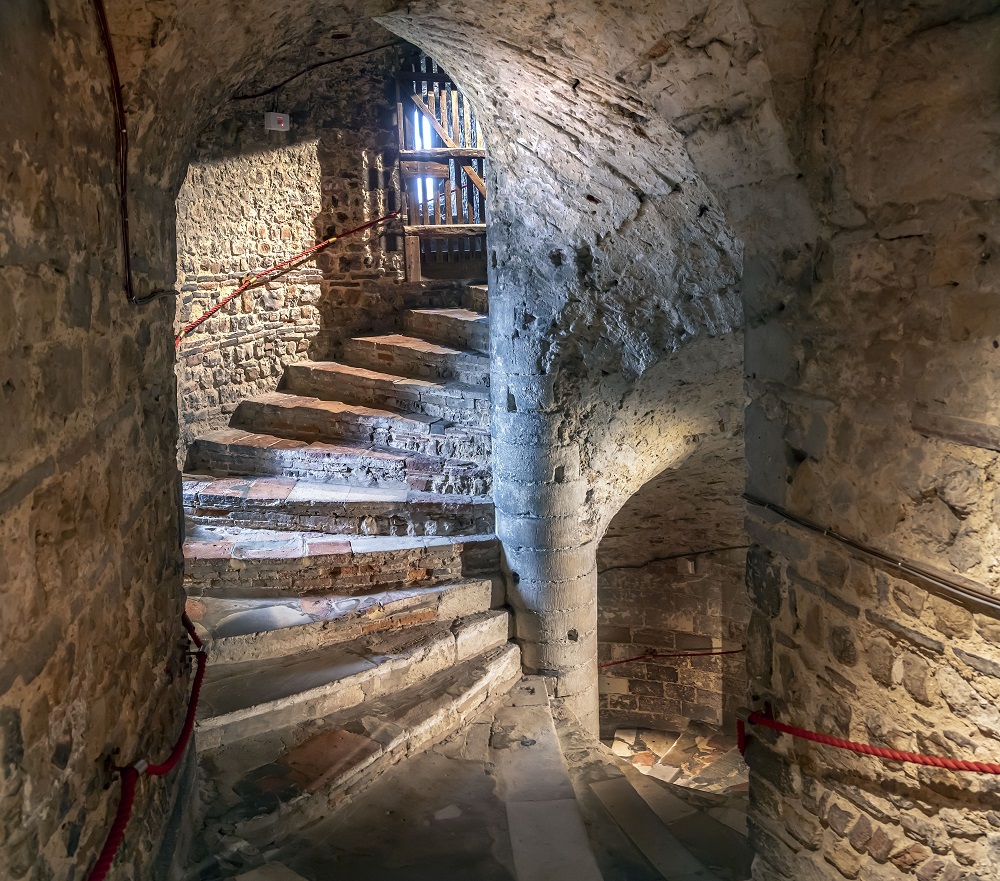This detailed image captures the ancient interior of what appears to be a stone tower or dungeon. Prominent in the scene are the weathered stone walls, predominantly brown and grey, showcasing intricate stone marks and patterns. Central to the image is a spiraling stone staircase, winding its way from the lower left upward to the right center. The stairs are highlighted with shades of brown and are accompanied by a handrail, with portions featuring accents of red rope. A notable feature is a dug-out stone seating area embedded into the rock walls, offering a place to rest. At the pinnacle of the staircase sits a wooden gate, adjacent to which a distinctive white and orange switch can be seen. The overall ambiance exudes antiquity and mystery, suggesting a structure that might once have served as a castle dungeon or clandestine hideaway.